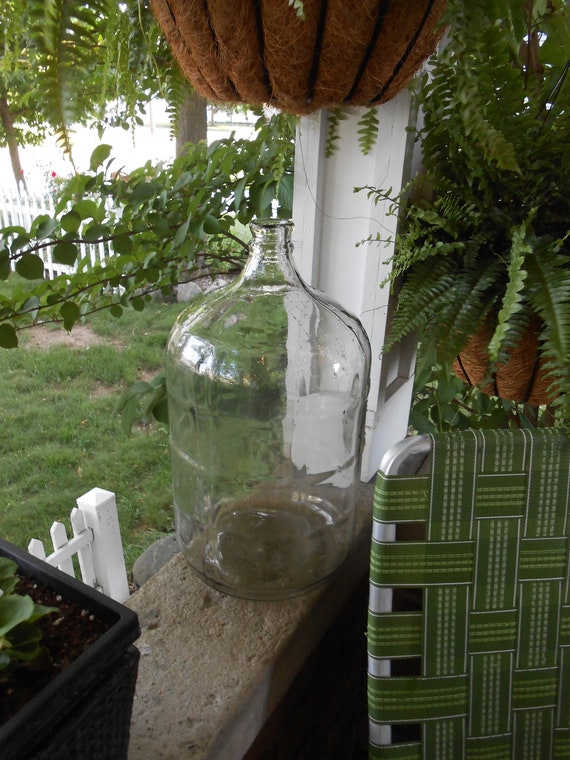This photograph captures a serene garden view from a porch. A gallon-size glass jug rests prominently on a cement wall, complemented by a nearby potted plant with green leaves peeking out. To the side, an old-fashioned aluminum lawn chair featuring woven green fabric adds a nostalgic touch. Above, a hanging basket, likely filled with plants, contributes to the lush ambiance. The scene extends to reveal a white picket fence and verdant grass, with various other plants, including ferns, enhancing the garden's rich greenery.